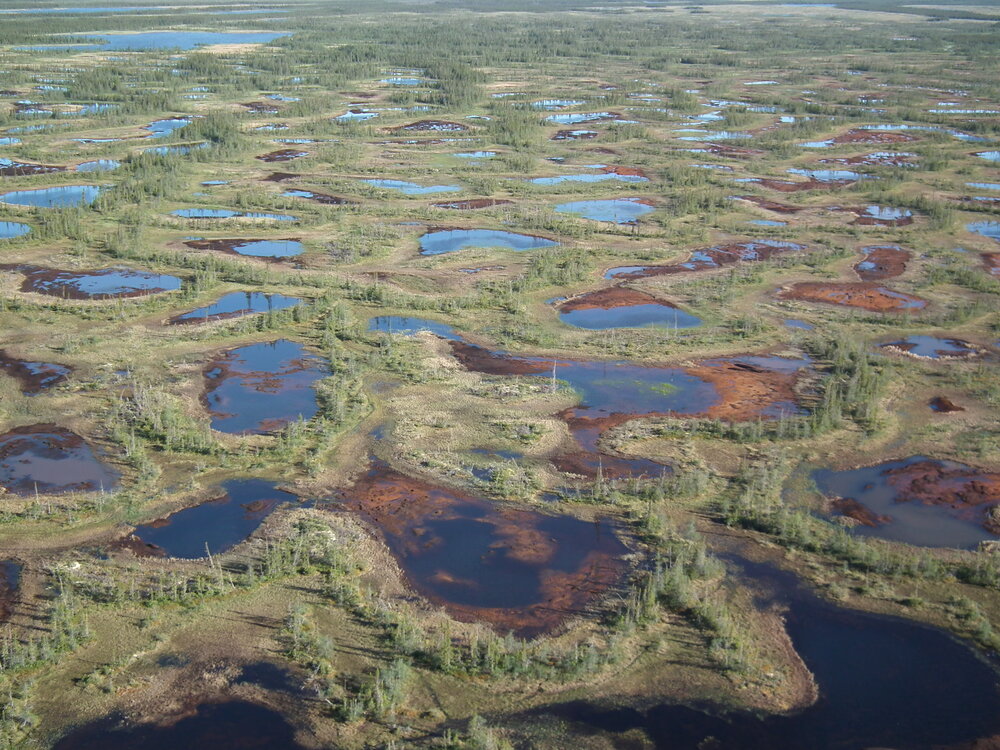This aerial image displays a sprawling marshland characterized by a mosaic of water bodies and earthy terrains. Multiple ponds, ranging from small to moderately large, punctuate the landscape. These water bodies feature variably colored shores, from brown and tan to copper and dark blue hues, indicative of different dirt types and organic materials. Algae and mud seem to inhabit some of these pools, lending them a murkier appearance.

The land between the ponds consists of patches of dry soil, scattered bushes, and trees. Closer examination reveals a variety of plant life: some areas with sparse, dry grass transitioning into denser, greener vegetation further out. The trees, appearing small from this high vantage point, are sprinkled across these patches of land, contributing to the scene's natural, untamed quality.

The entire frame is filled from top to bottom and side to side with this untouched marshy expanse, devoid of human presence, roads, or structures. The larger body of water in the upper left-hand corner serves as a focal point, enhancing the sense of wilderness and isolation. Overall, the image captures the intricate, unorganized beauty of a remote marshland ecosystem.